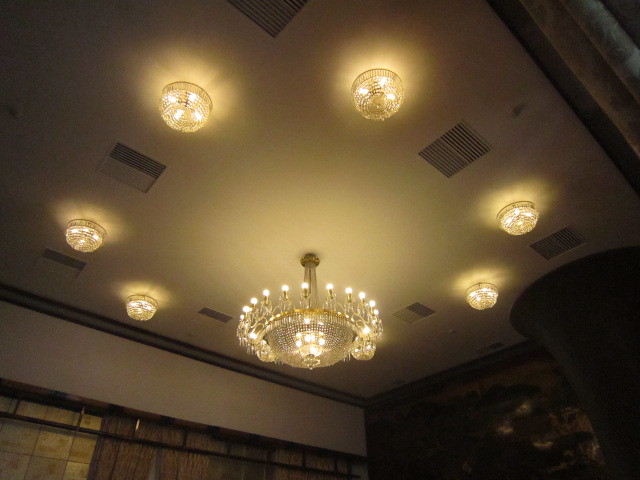This image captures the intricate ceiling of a room adorned with Chinese traditional style murals that depict landscapes in blacks, greens, golds, and whites. The ceiling itself, painted white, features an array of lighting fixtures. Dominating the center is a dazzling chandelier that sits close to the ceiling, adorned with candle-like bulbs encircling its perimeter. Crystal chains cascade toward its disco ball-like base, adding a touch of elegance. Surrounding this centerpiece are eight flush-mounted lights that match the chandelier in style and color, forming a geometric arrangement. These fixtures provide a cohesive aesthetic, while vents, presumably for heating, are interspersed across the ceiling. This close-up photograph offers a detailed view of the ceiling’s sophisticated lighting and decorative elements.